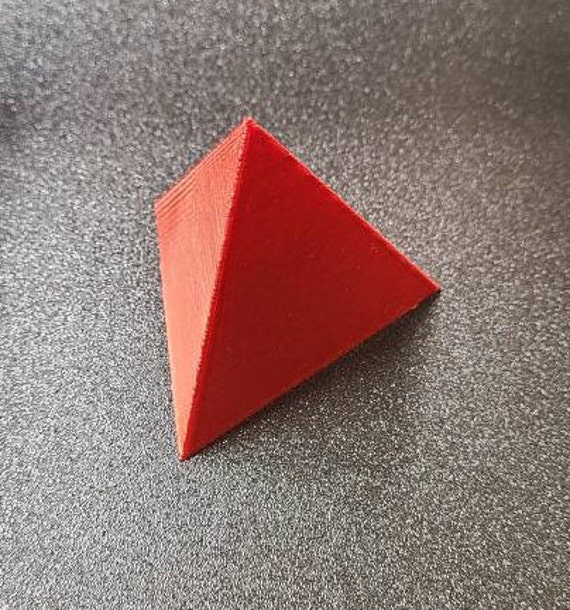The image is a vertical, color photograph featuring a close-up of a small, bright orange pyramid constructed from a foam or plastic-like material. The pyramid, which appears to have two visible faces, is lying on its side on a speckled gray surface, possibly made of linoleum or stone. The surface has a textured pattern with white and gray spots, and the lighting creates varying shades of gray, becoming darker towards the top of the image. The pyramid, a central focal point, is the only object in the otherwise simple and unembellished photograph. The overall effect of the lighting and shadows creates a realistic impression, suggesting that the image might be computer-generated.